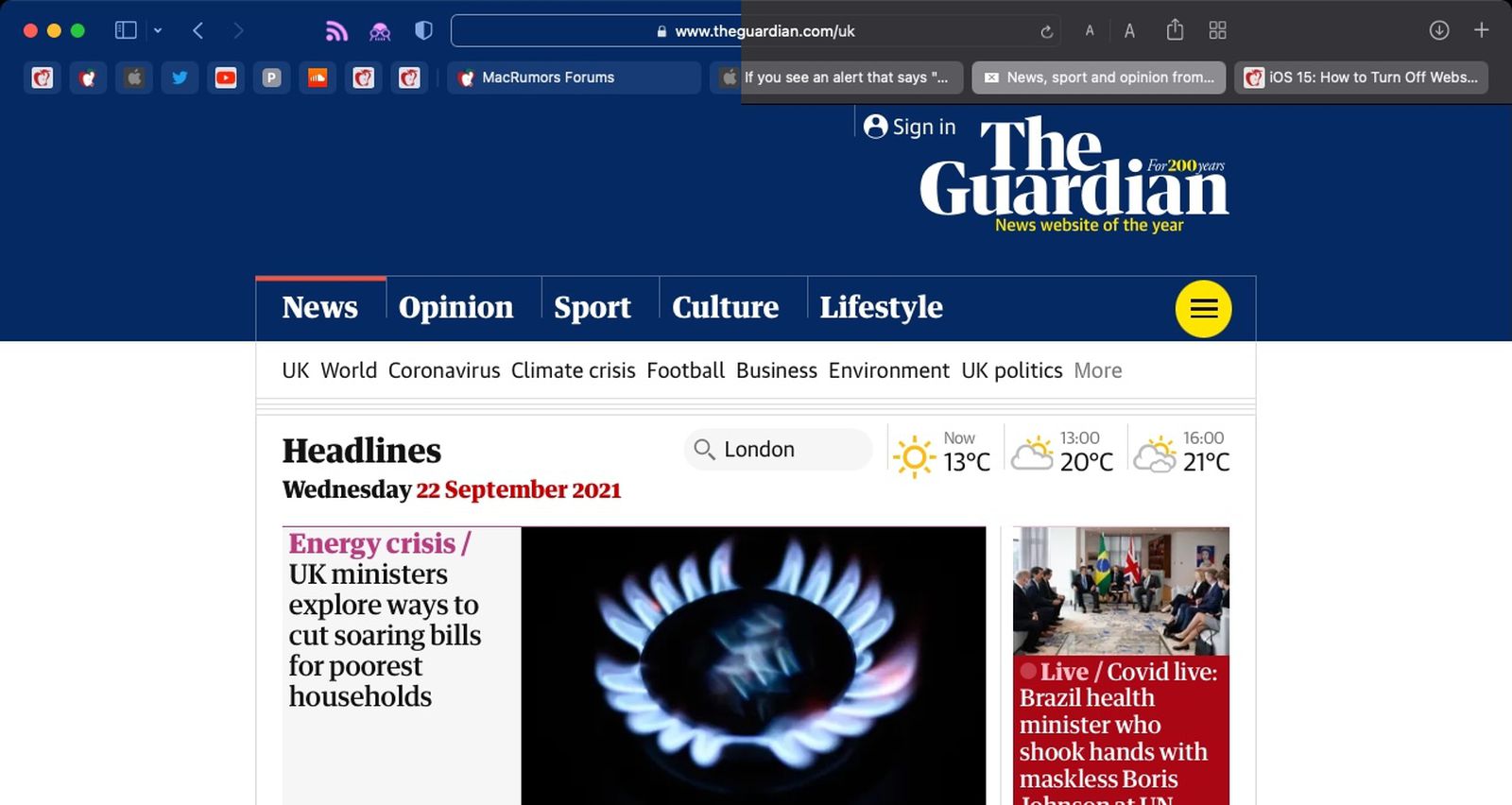This digital image showcases the interface of The Guardian's news website, acclaimed as the "News Website of the Year." The top of the page is highlighted by a prominent thick navy blue border displaying the site's title in bold. The left side of the image is crowded with various thumbnails, incorporating a mix of colors including red, blue, and a noticeable Apple logo.

On the right side, notifications pop up, including updates like "News, Sport, and Opinion from an iOS" and a prompt on "How to Turn Off Webs." Beneath these alerts, the navigation menu lists categories such as News, Opinion, Sport, Culture, and Lifestyle. Further subcategories include UK, World, Coronavirus, Climate Crisis, Football, Business, Environment, UK Politics, and more.

The headline section beneath the menu specifies the date: Wednesday, the 22nd of September 2021. Weather information for London is provided, detailing that at 13:00, the temperature is 13°C, expected to rise to 20°C by 13:00 hours and 21°C by 16:00 hours.

The central content focuses on the energy crisis, highlighting efforts by UK ministers to alleviate soaring energy bills for the poorest households. This segment is accompanied by an illustrative icon depicting a flame, symbolizing a burner, and is tagged with the label "Live."

Additionally, there is a live update about COVID-19, mentioning the Brazilian Health Minister who had an encounter with a maskless Boris Johnson.